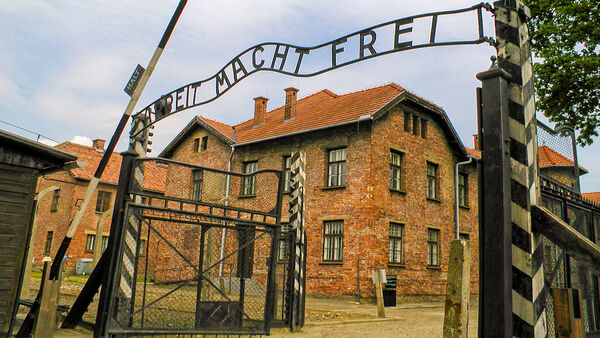The image depicts the main gate of Auschwitz, the infamous Nazi concentration camp where Jews were imprisoned during the Holocaust. Prominently displayed at the top of the entry gate is the notorious phrase "Arbeit Macht Frei," written in a foreign European language, which translates to "Work Sets You Free" in German. The scene shows a black and white gate that swings up and down to allow cars in, accompanied by a metal chain-link fence that stands open. Beyond the gate, there are several large brick buildings with red tile roofs and chimneys, each featuring about four windows per side. The photograph, with its notably saturated colors, captures a clear, light blue sky and a tree with visible leaves on the right side. The setting is framed by a sense of historical gravity, evoking the somber memory of the atrocities committed within the camp.